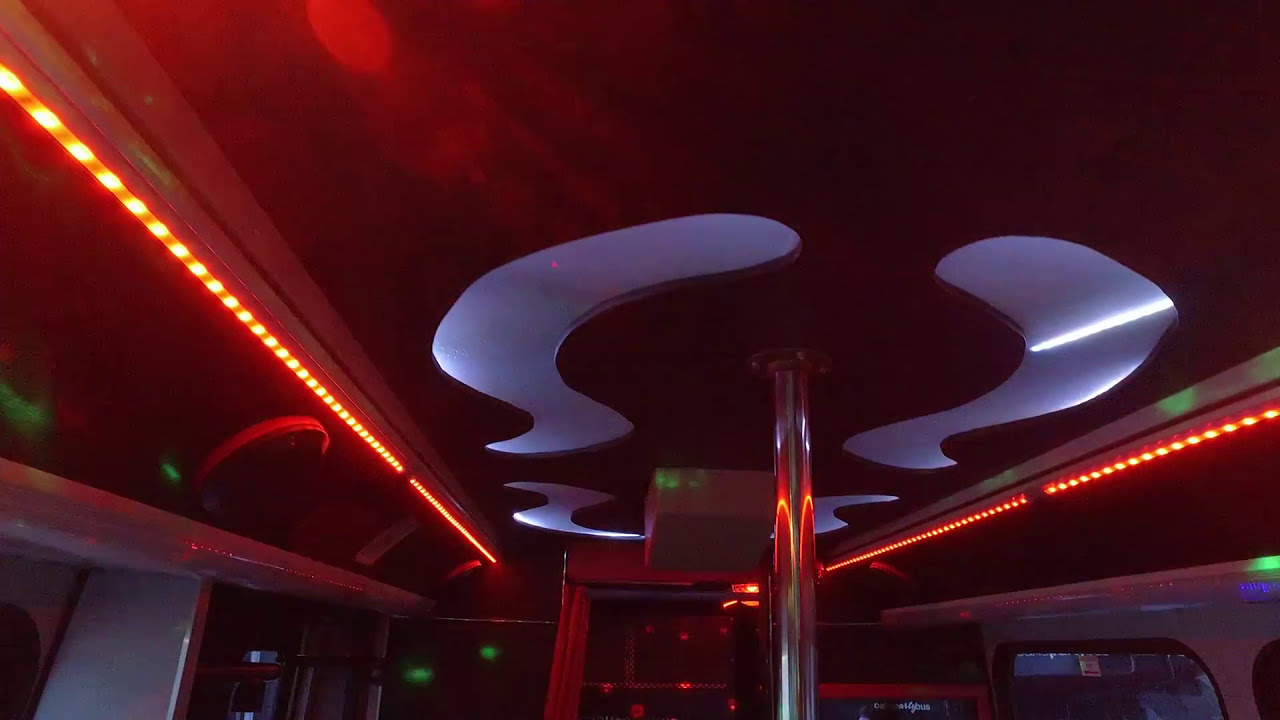The image primarily showcases the ceiling of what seems to be a small, possibly public space or interior of a vehicle, likely a party bus. The ceiling is predominantly black, with distinct touches of color and light. Along the left and right sides, there are glowing red LED lights arranged in strips. A shiny silver pole descends from the center, surrounded by curvy, abstract cutouts that are light blue in color. To the left of the pole, a white box is attached to the ceiling, adding to the intricate design. The very tops of rounded square windows beneath the ceiling can also be seen, suggesting the setting might be within a vehicle or a confined space. Reflective and ambient lighting, including hints of light green and off-red hues, enhance the dark and somewhat mysterious ambiance of the scene.